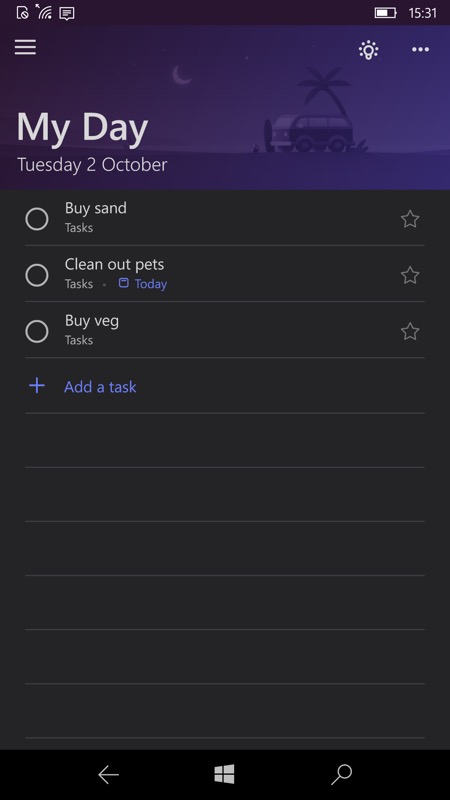This is an intricate screenshot of a phone displaying a to-do list application. At the top of the screen, the phone's status bar shows the current time as 3:31 PM, along with the battery life and signal strength indicators set within a black background. Below this, there's a visually appealing banner featuring a blue and purple gradient with a shadowy silhouette of a Volkswagen van driving under moonlight next to a palm tree. The date is clearly marked as Tuesday, October 2nd.

Immediately below the banner, the application interface is organized into multiple tasks. The first task is displayed within a black box labeled "task," and includes a star icon on the right for marking it as important. The task description reads "Clean out pets," highlighted with a 'Today' tag in blue.

The second task on the list, also within a black box and labeled "task," is "Buy vegetables" accompanied by a star icon on the right.

A blue 'plus' sign followed by the text "Add a task" indicates where new tasks can be added to the list. 

At the very bottom of the screen, the phone's navigation bar presents the familiar icons: a back arrow, a home button, and a search icon. This completes the well-organized layout of the to-do list application on the user's phone.